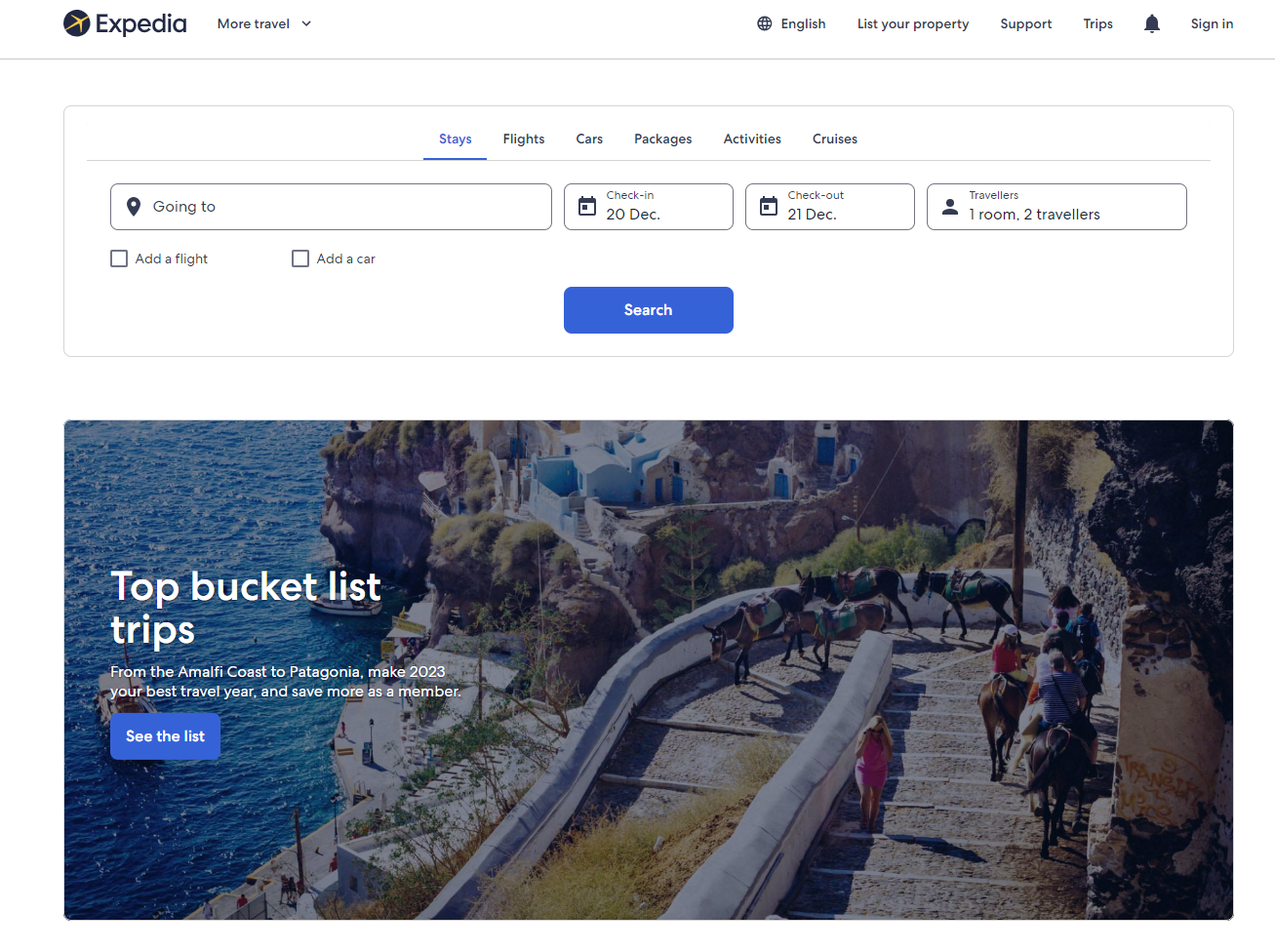"Top Bucket List Trips for 2023"

In this captivating image, you'll see an enticing travel advertisement with a detailed layout designed to inspire wanderlust. Positioned on the left, the headline "Top Bucket List Trips" is presented in bold white text. Below this, a subheading in smaller white font reads, "From the El Merfri coast to Patagonia, make 2023 your best travel year and save more as a member." 

Central to this composition is a blue rectangle with the call-to-action "See the list" prominently displayed in white lettering. The background of the image features a breathtaking scene of a group of people on horseback, navigating a winding staircase that curves to the left and then descends. The landscape includes a picturesque view of land dotted with trees and bordered by a tranquil body of water to the left.

Above this scenic depiction, the rest of the image transitions to a clean white background. Here, you'll find a blue search bar with selectable options: “Going to,” followed by “Check-in,” “Checkout,” and “Travelers, one room, two travelers.” Below the search bar, there are two additional boxes labeled "Add a flight" and "Add a car."

On the top-left corner, the name of the website, Expedia, is displayed. Adjacent to this, a tab labeled "More travel" is visible along with a navigation menu comprising five options: “English,” “List your property,” “Support,” “Trips,” and a notification bell icon, followed by “Sign in.” All text in the navigation menu is presented in black lettering, neatly rounding out the visual design of the image.

This ad layout not only provides a visually appealing travel scene but also integrates functional elements for seamless user interaction.